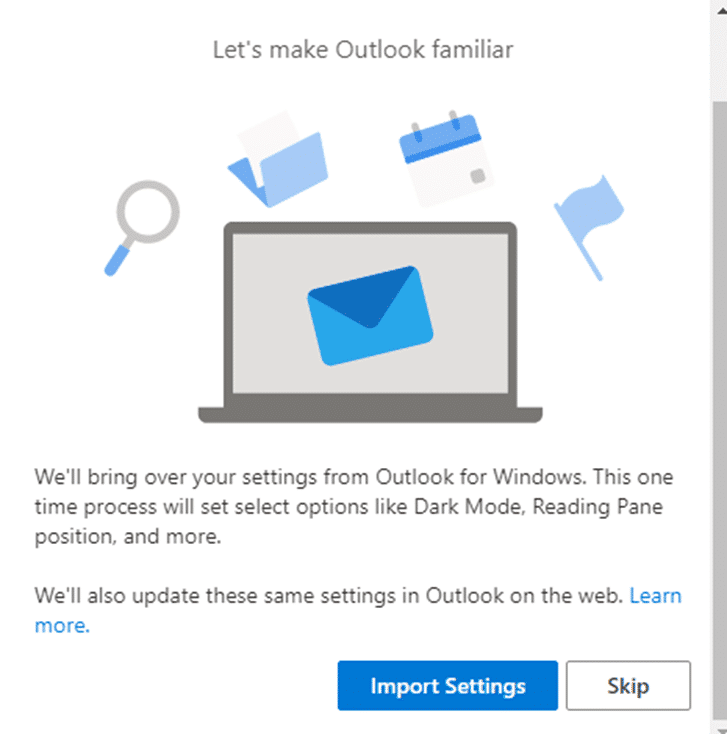Against a pristine white background, this image appears to be a web page centered around making Outlook more familiar to users. At the top center of the page, bold black text reads, "Let's Make Outlook Familiar." Below this header, an open laptop is illustrated in a cartoonish, gray style, displaying a screen with a prominent blue envelope. The envelope sports a darker blue flap contrasted by a lighter blue body.

Hovering around the laptop are various icons: on the left, a magnifying glass with a gray lens and a blue handle; to the right of this, an open blue folder with a white sheet of paper emerging from it; next, a white electrical plug with a blue cap and dual gray prongs. Further to the right and slightly lower, almost beside the laptop, is a simple blue flag icon.

Beneath the laptop, black text informs users: "We'll bring over your settings from Outlook for Windows. This one-time process will set select options like dark mode, reading pane position, and more." Below this, additional text states, "We'll also update the same settings in Outlook on the web," ending with a blue hyperlink that says "Learn more."

At the bottom-right corner of the page, there are two action bars. The first bar is blue with white text that reads "Import settings," while the second bar is white with black text that says "Skip."